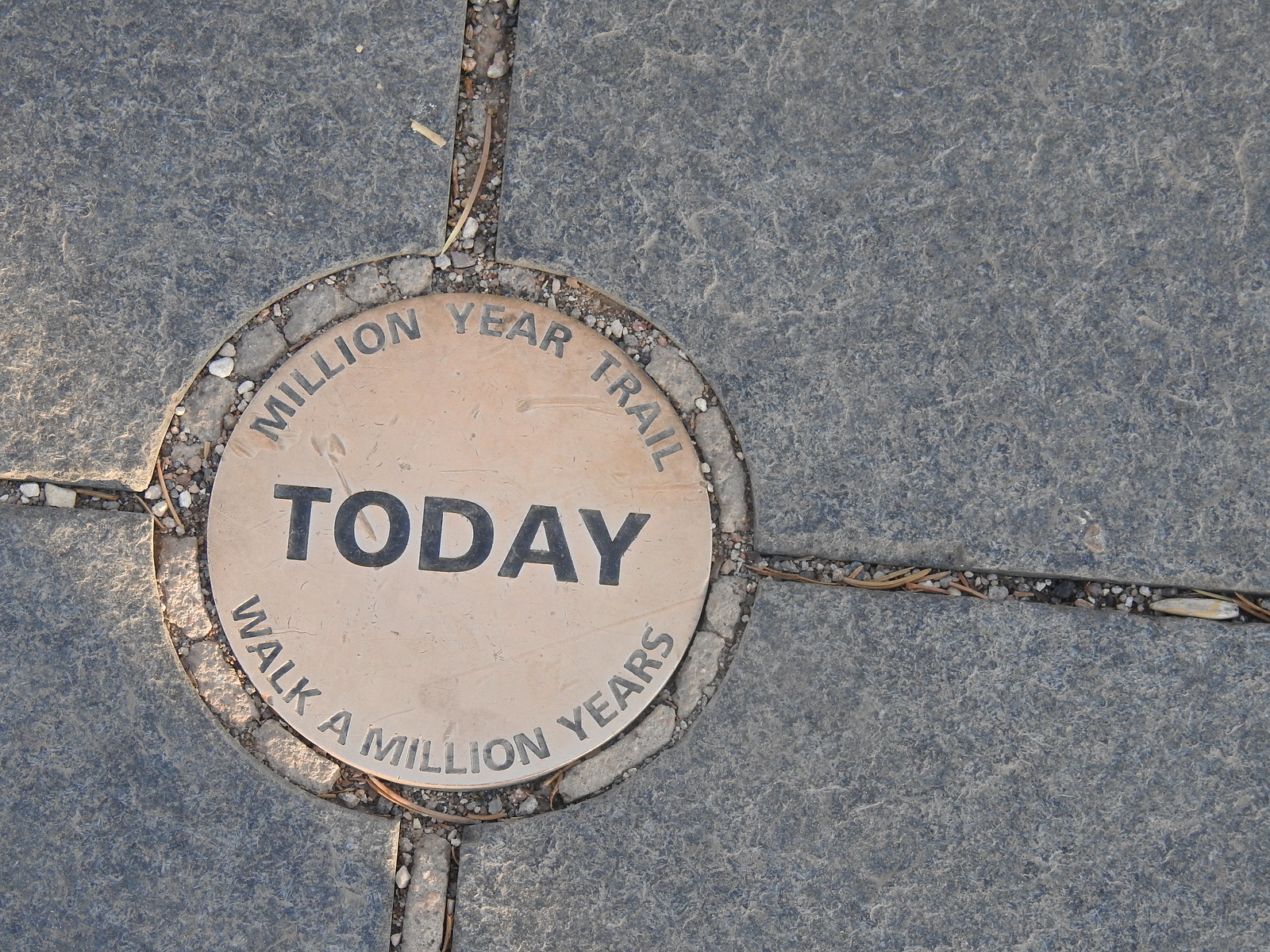The image showcases a round, worn engraving set into a black and white marble background, likely part of a sidewalk. The engraving is centrally placed, with lines radiating from it in all four cardinal directions, giving it a circular, slightly old appearance. In the circle's interior, the background is light, possibly pinkish. At the top of the circle, in light black lettering, it reads "MILLION YEAR TRAIL," while the center prominently features the word "TODAY" in big, bold black letters. At the bottom, it says "WALK A MILLION YEARS" in worn black lettering. Surrounding the engraving, debris such as pebbles and leaves are visible in the cracks between the tiles that comprise the walkway.